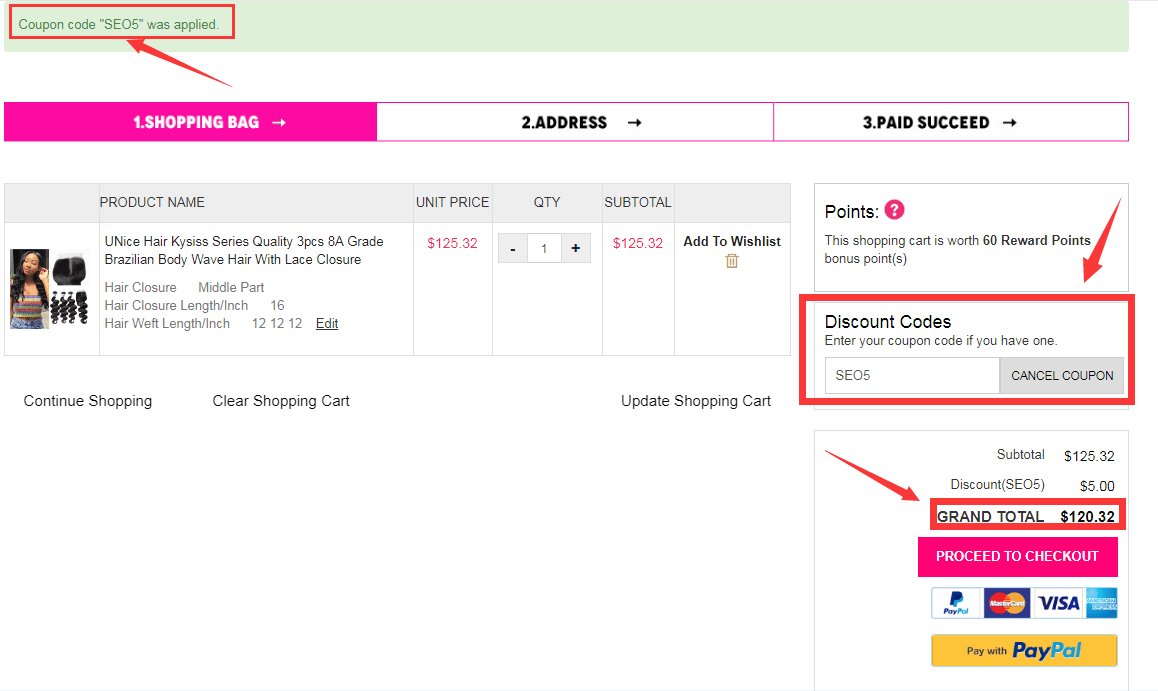The screenshot features an online shopping cart page filled with detailed elements and options. Dominating the top-left corner is a red-boxed area with a green background and darker green text, indicating that the coupon code SE05 has been successfully applied. The page is titled "Shopping Bag" in white text against a pink background, marking the current step in the checkout process. Adjacent to this are steps indicating the progression: "2. Address" and "3. Paid," signifying the subsequent stages.

Displayed prominently is the product listed for purchase: "Unis Hair Kindness Series Quality 8A Grade Brazilian Body Wave Hair with Lace Closure (3-piece set)." The unit price is highlighted in bold red text as $125.32. The quantity selected is one, leading to a subtotal of $125.32. Users have the options to add the item to their wish list or delete it, symbolized by a little trash can icon. Below the product summary are options to "Continue Shopping," "Clear Shopping Cart," and "Update Shopping Cart."

Additional details include a points summary, revealing that the shopping cart accrues 60 reward points. Under "Discount Codes," the applied SE05 is shown again within a red box, with an option to enter another coupon code or cancel the existing one. The financial breakdown lists an item subtotal of $125.32, a $5 discount courtesy of the SE05 code, leading to a grand total of $120.32.

Finally, the page provides payment options, including buttons for "Proceed to Checkout," "PayPal," "MasterCard," "Visa," and "American Express." There's also a reiterated option to pay specifically with PayPal. The detailed and organized layout presents a clear and comprehensive view of the shopping cart's contents and payment procedures.